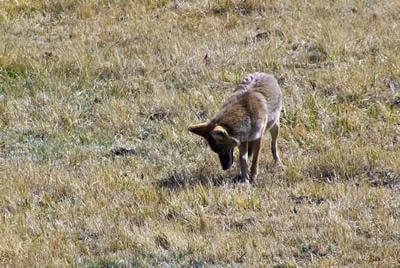The photo captures a medium-sized coyote positioned in the center of a vast grassland. The coyote, with a sharp angular nose and fur primarily in shades of gray and brown, stands in a patch of predominantly yellowed, sparse, and dead grass, although some areas show hints of green. Its body, healthier-looking and possibly indicating a well-fed or pregnant state, features a white underside and inner ears. The coyote is intently staring down at the ground, likely hunting near some visible gopher holes. A stark black shadow is cast on the grassy terrain, echoing the coyote's form. The sunlight illuminates its body, but its face remains shadowed, adding to the overall enigmatic atmosphere of the scene.